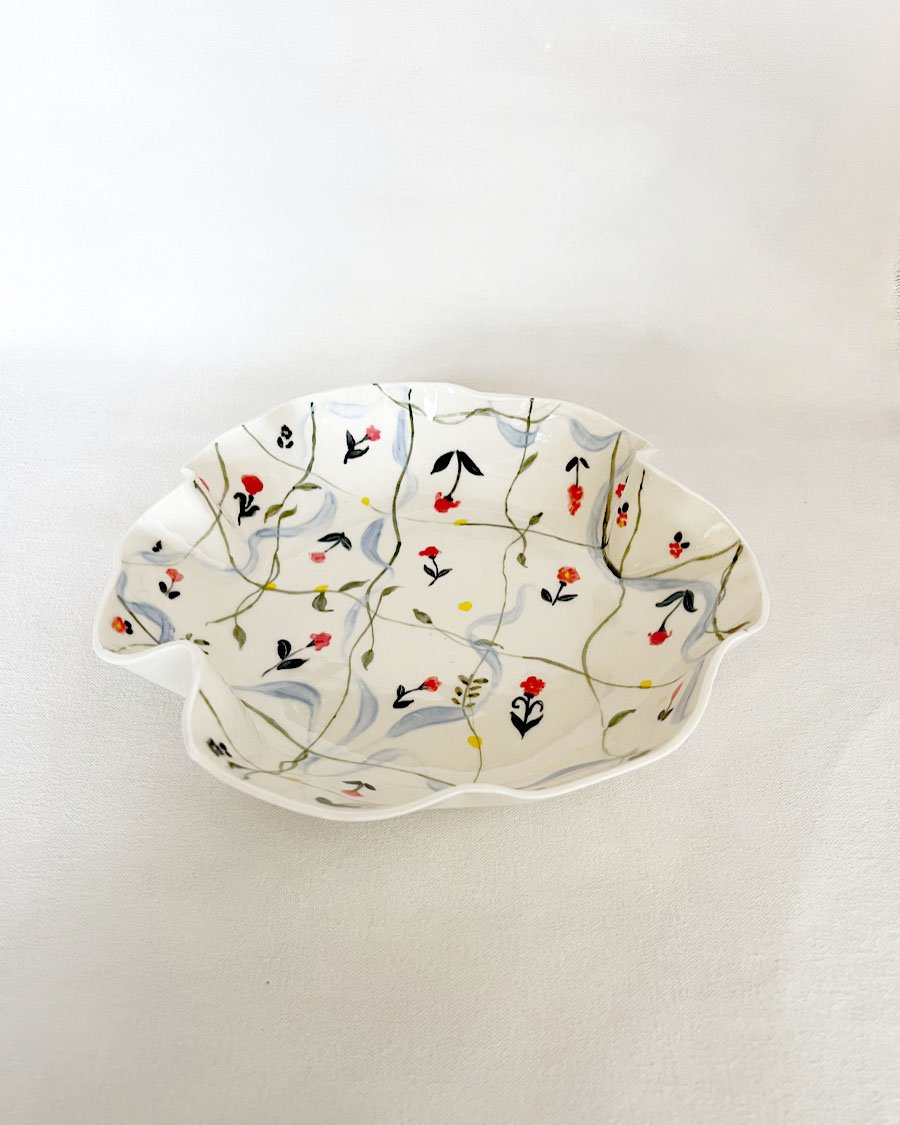This photograph depicts a uniquely shaped ceramic bowl, resting on a mostly white, slightly tarnished rectangular background. The bowl, predominantly white, features an irregular circular form with wavy or folded edges akin to a pie crust, creating a visually appealing ripple effect. Inside the bowl, a detailed floral pattern stands out. This pattern consists of crisscrossing vine-like grids in green, forming odd-shaped squares, each housing a delicately painted flower. The flowers predominantly display bright red petals with black stems and some pink hues. Additionally, the intricate interior design showcases gray wavy patterns and swirls, enhancing the bowl's artistic appeal. The scattered floral elements, comprising red blooms and green vines with sparse leaves, contribute to the bowl's elegant and charming aesthetic.